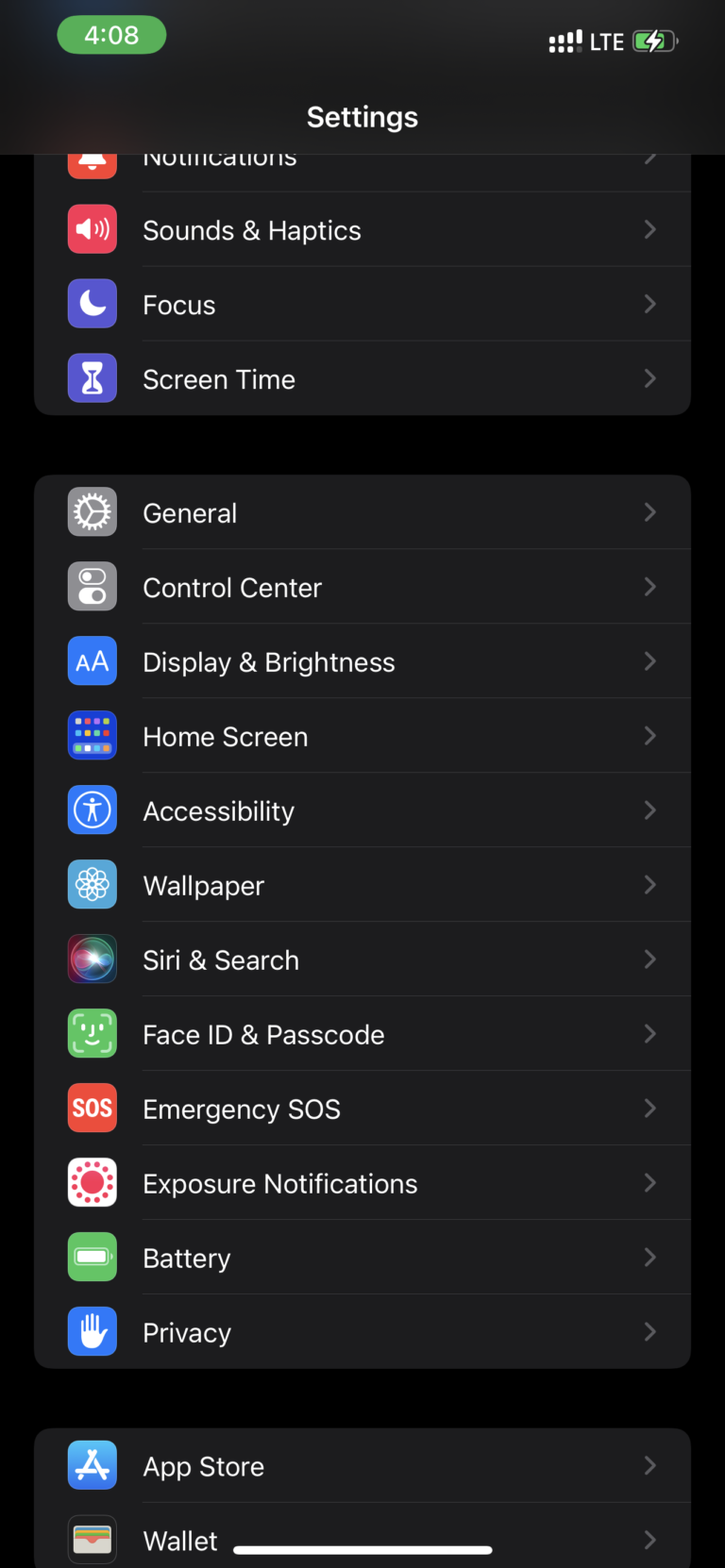This screenshot, taken from an iPhone in dark mode, prominently features the device's settings menu. At the top left corner, the time is displayed as 4:08 within a green oval-shaped icon with white text. To the right, the screen indicates that the user is connected to an LTE network. The battery icon shows that the phone is not fully charged but actively charging, as signified by the lightning bolt symbol.

Beneath the status bar, the word "Settings" is displayed in white text as the header. The menu items are listed in white text on a dark grey background, beginning with "Sounds & Haptics," followed by "Focus," "Screen Time," and then "General." The list continues with "Control Center," "Display & Brightness," "Home Screen," "Accessibility," "Wallpaper," "Siri & Search," "Face ID & Passcode," "Emergency SOS," "Exposure Notifications," "Battery," and "Privacy."

At the bottom of the screenshot, a new section begins with "App Store" and "Wallet," marking the end of the visible portion of the settings menu.